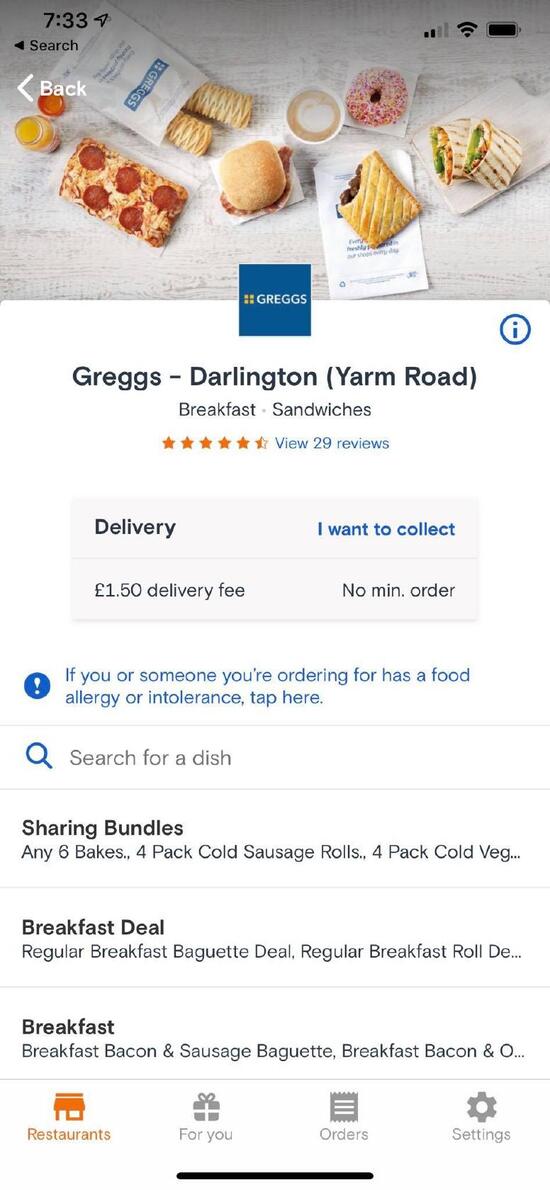The screenshot image from the smartphone provides several details. At the very top of the image, the status bar displays the time as 7:33, a Wi-Fi signal is present, and the battery icon indicates a full charge on a black background. Below this, we see a photograph depicting a variety of treats: breadsticks, a square slice of pizza, a small chicken sandwich, an assortment of pies, a burrito-type sandwich cut in half, a donut, and a beverage that appears to be either hot chocolate or flavored coffee.

Scrolling further, the image shows the name "Greg's Darlington" with the location specified as "Yarm Road" in parentheses. The establishment offers breakfast and sandwiches and has received 4.5 stars based on 29 reviews. Delivery services are available with a $1.50 fee, and there is no minimum order requirement. A blue-colored notification suggests tapping for information regarding food allergies or intolerances. 

Additionally, the screenshot presents an option for ordering sharing bundles, including combinations like any six bakes, four cold sausage rolls, and four cold vegetable options (only "veggie" is fully visible).